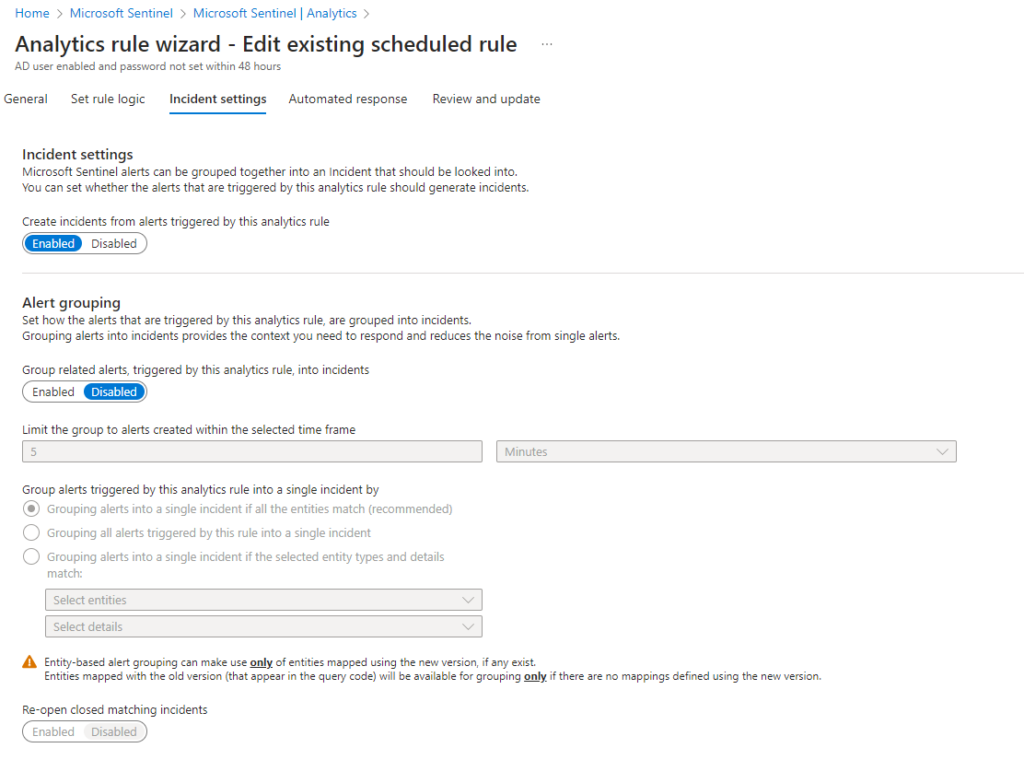This screenshot captures a webpage from a Microsoft-related site, specifically within the Microsoft Sentinel platform. The navigation path at the top left traces back through several tabs, sequentially labeled: Home, Microsoft Sentinel, and Microsoft Sentinel Analytics. The current page is titled "Analytics Rule Wizard - Edit Existing Schedule Rule," which is prominently displayed in bold black text.

Beneath this title, there is a series of tabs for different sections: General, Set Rule Logic, Incident Settings (the highlighted tab), Automated Response, and Review and Update. Under the 'Incident Settings' tab, there is an option to enable or disable the creation of incidents from alerts triggered by the analytics rule. Another section labeled 'Alert Grouping' allows users to group related alerts, with a toggle to enable or disable this feature, which is currently set to disabled.